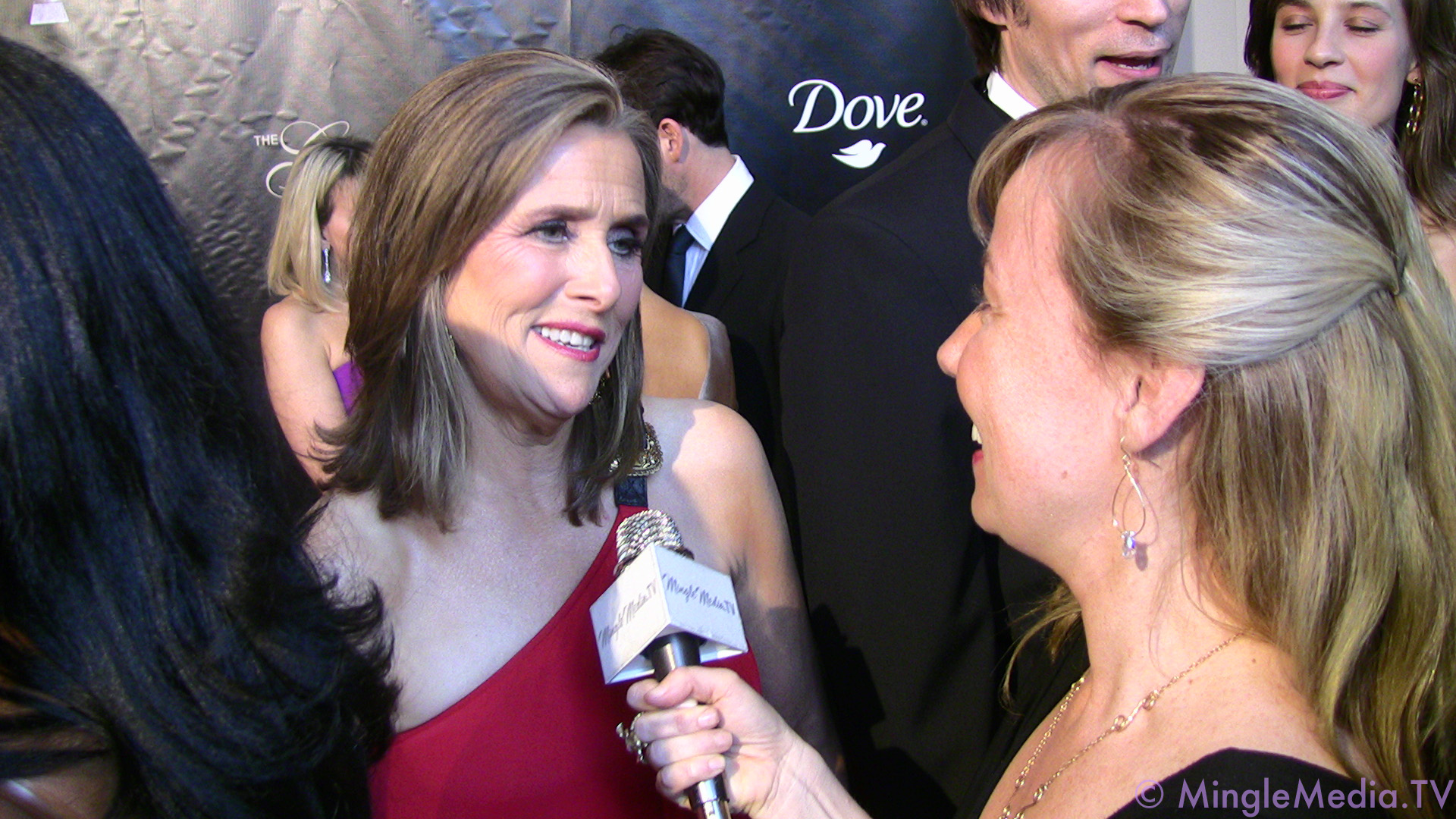The photograph captures a lively event with numerous attendees, set against a backdrop featuring the logo and name of the Dove company. In the foreground, two central figures draw immediate attention: a middle-aged woman in a red sleeveless gown with long brown hair, being interviewed by another woman with blonde hair, who is holding a microphone encased in a white triangle. The interviewer, a white woman wearing a black dress adorned with earrings and a locket, stands to the right of the image.

Surrounding these focal characters are several other attendees, their faces partially visible. To the left, a woman's hair is just visible, while in front of the banner stand two more individuals, a male and female. The male, dressed in a black suit, white shirt, and black tie with dark hair, is somewhat obscured by two women—one with only the back of her head visible and another in a purple off-shoulder dress with blonde hair. In the right corner of the image, partially visible, are more attendees, including a man in a black suit and another female.

The crowd's configuration and varied attire, coupled with the corporate banner, suggest a formal gathering, perhaps a corporate event or gala. The image also features a visible copyright source in the bottom right corner, tagged as MingleMedia.tv.